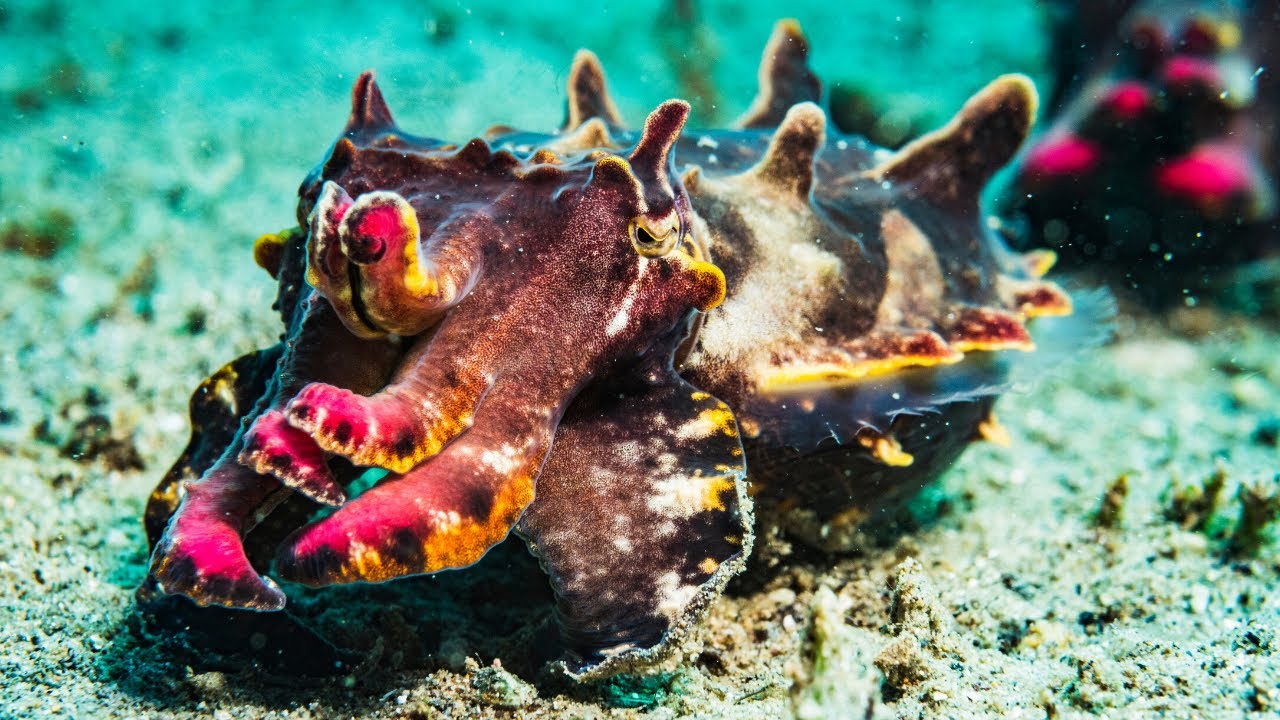This detailed underwater photograph captures the intriguing scene of a shelled sea creature, possibly a sea snail, set against a sandy and gravelly ocean floor. The creature is prominently displayed in the foreground, showcasing a vibrant and varied color palette of hot pink, yellow, dark purple, beige, orange, red, and black. Its distinctive features include six spiky horns protruding from its head and back, which resemble a mountainous landscape. The creature has black eyes with gold outlines, adding to its striking appearance. Surrounding it, the base is a blend of tan and cyan hues, with small goldish objects sticking up from the sand. The blurred background reveals another similar creature with bright pink and black coloring, accompanied by hints of green foliage and bubbles, suggesting an underwater environment. However, the presence of a reflection on the right side might indicate that the creature is actually within an enclosure, well-lit for detailed observation.